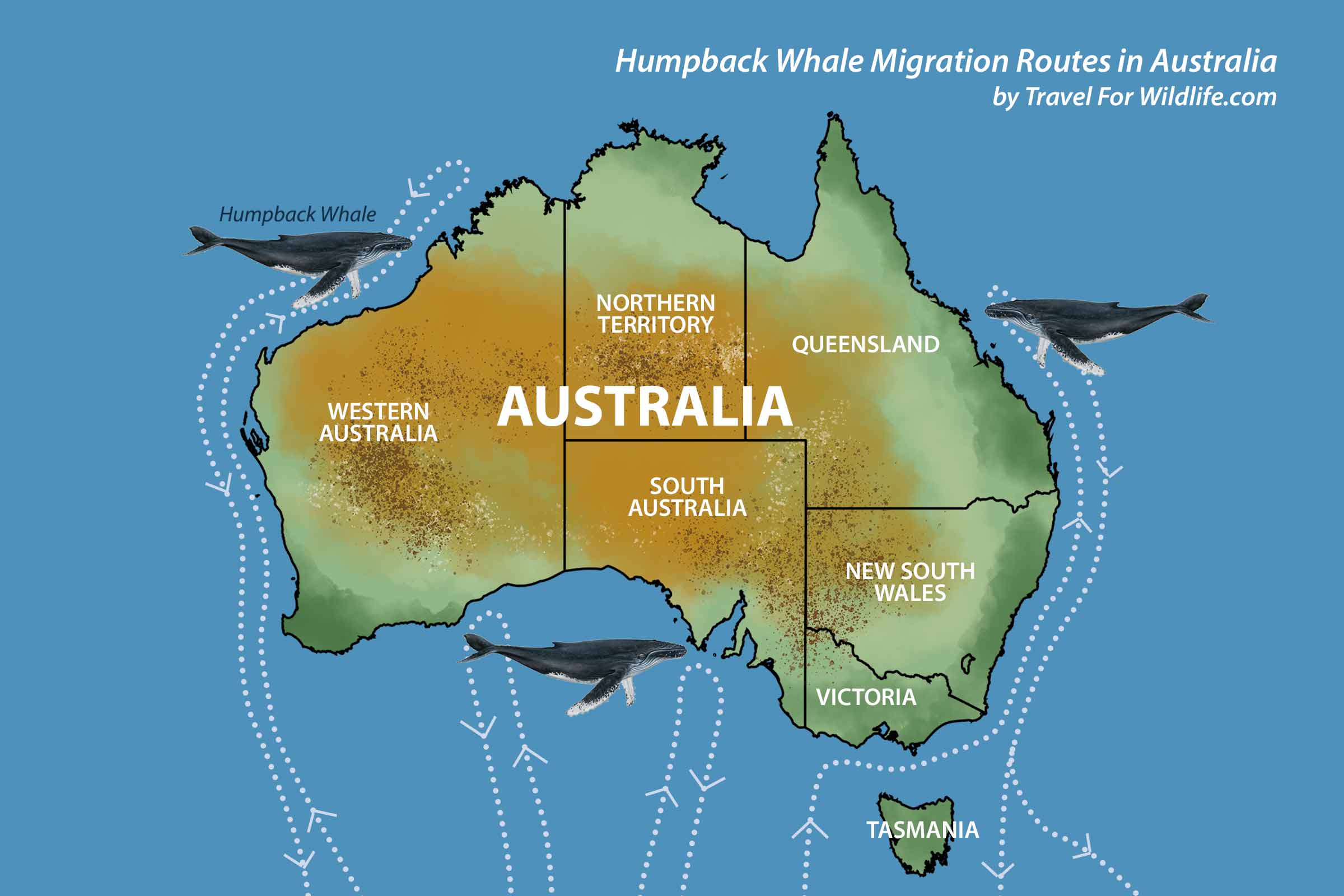This detailed artist's sketch map, set against a light blue oceanic background, illustrates the humpback whale migration routes in Australia, courtesy of travelforwildlife.com. The Australian continent is depicted in shades of brown and green, bordered in black, with distinct sections marked for Western Australia, Northern Territory, South Australia, Queensland, New South Wales, Victoria, and the island of Tasmania. The map features three humpback whales near key locations: just north of Perth in Western Australia, near South Australia in the inlet, and on the upper right side of Queensland. Each whale is connected to dotted migration routes that trace their paths northward and back southward. The map foregrounds the importance of these migratory patterns with precise directional arrows, placing particular emphasis on the regions traversed by the whales.